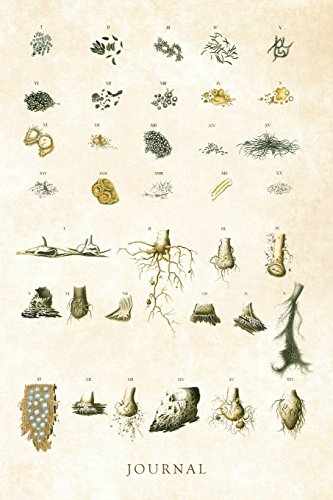The image is a vertically rectangular print piece set against a mottled light brown, aged-looking background with no border. It appears to depict scientific illustrations, arranged in six rows, each containing about five or six detailed sketches. These illustrations predominantly feature various seeds at the top and transition to roots, stems, and bulbs towards the bottom, effectively showcasing different stages of plant growth. Most of the images are rendered in dark yellow or dark gray colors. Each illustration is labeled with small, somewhat blurry numerals, possibly Roman numerals. The word "JOURNAL" is prominently displayed in all capital black letters at the bottom of the piece. The numbers and labels, while present, are difficult to read, indicating detailed annotations for each plant part.